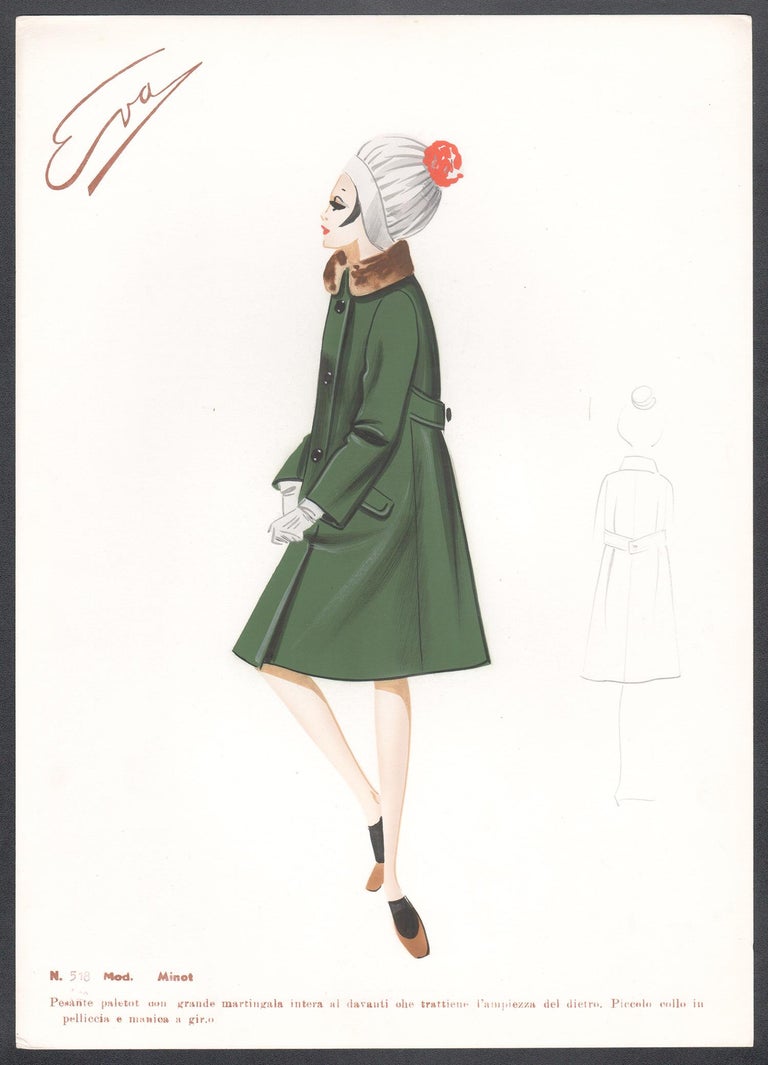The image is a detailed color artwork portraying a woman named Eva, as indicated by the word "EVA" sketched at the top left corner. Eva is elegantly dressed in a cream pea coat with a fur collar, resembling a skirt at the bottom, which has long sleeves and big black buttons. Complementing her ensemble, she wears white gloves, black socks, and small brown shoes. Her slender, pale legs and overall lithe appearance add to her graceful look. 

She dons a white winter hat adorned with a red accent or ball on top, from which a wisp of her dark black hair escapes. The background features a faint outline of another figure, adding depth to the portrait. The text "N518 Maud Minot" appears at the bottom in a brown font, written in a language that seems to be French or Italian. The entire image is set against a white background, enhancing the clarity and focus on Eva.